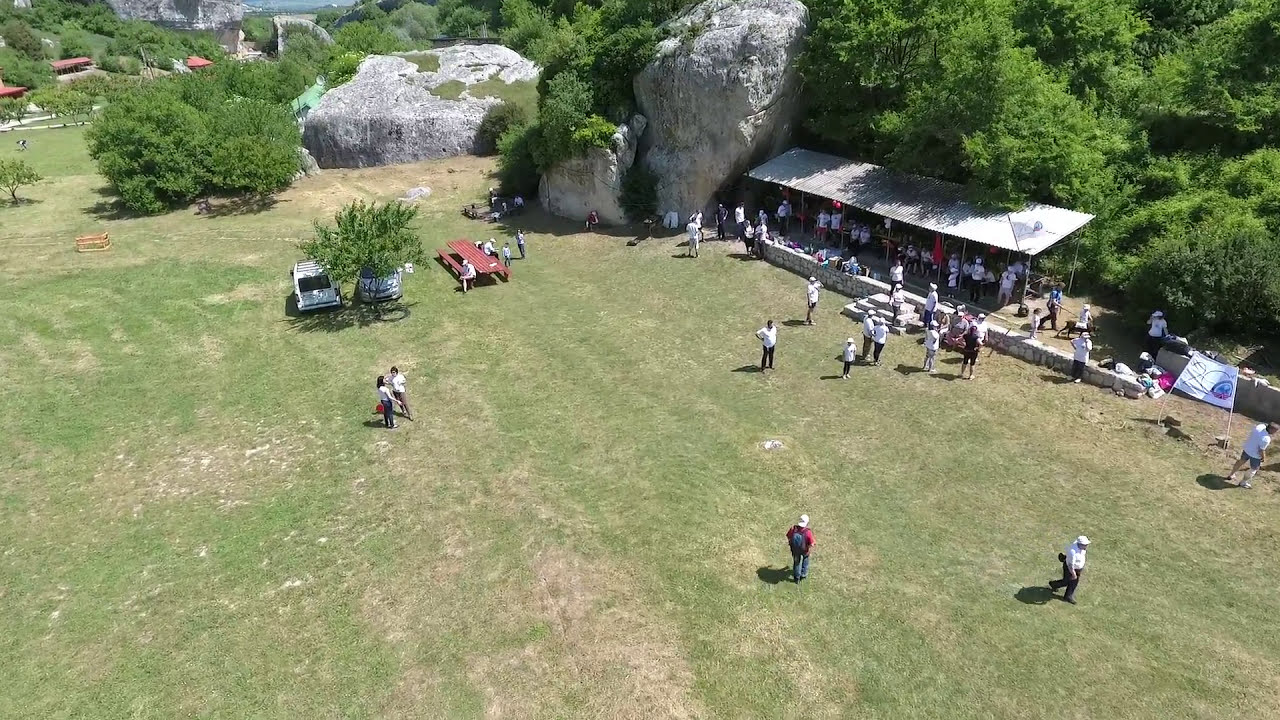The image is an aerial photograph of a large, sunlit open field that appears to be the site of a family get-together or party. The scene is set near a base of a mountain or hill adorned with humongous granite boulders, some reaching 30 to 40 feet tall. At the far right stands a metal canopy with a tin roof, under which individuals are gathered and seated at tables. A red picnic bench nearby accommodates more people. Vehicles, including an SUV and two minivans, are parked under the shade of sizable trees. Among the attendees, many are wearing white, some are mingling and talking, and others are possibly playing golf or simply enjoying the day. In the background, there are multiple huts or cabins with red tile roofs, adding to the picturesque, almost campground-like setting with lush green brush and towering trees surrounding the area.